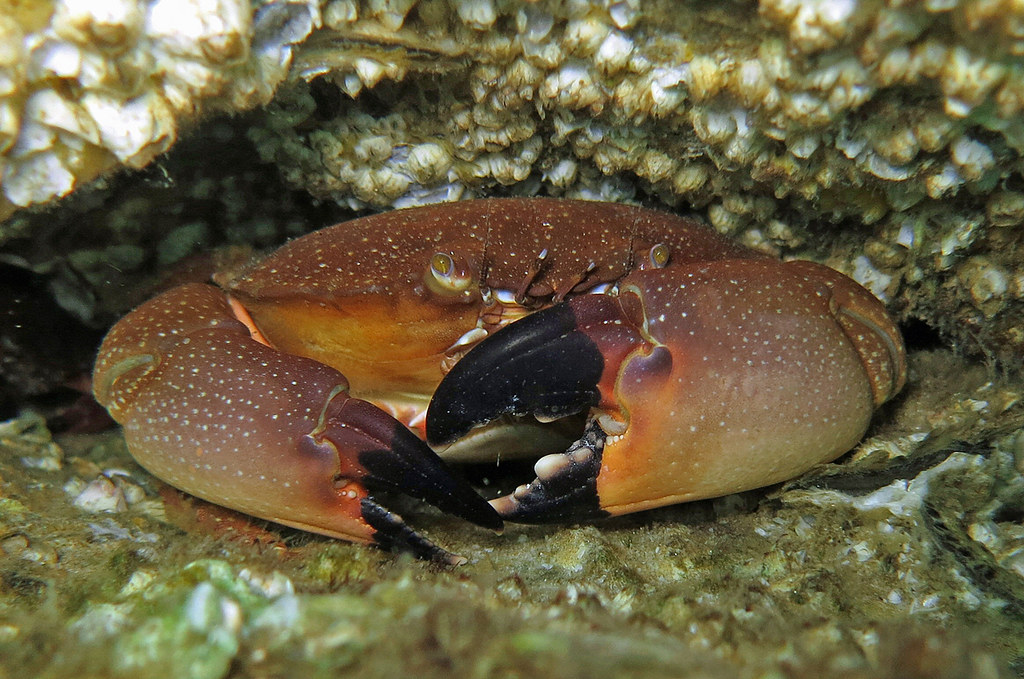This is a detailed close-up photograph of a stone crab hiding beneath a rock or coral underwater. The crab's overall coloration is a reddish-brown with a mottled pattern of white spots, giving it a muted and somewhat rugged appearance. Its claws are distinctively tipped in black, and the left claw is noticeably larger, open as if ready to grasp something, while the right claw is smaller, pointier, and more closed, resting on the bottom. The crab’s two brownish-gold eyes and paired brown antennae are visible, with the eyes peering out and giving it a grumpy expression. A small portion of the crab's mouth is visible, not entirely obscured by the left claw. The surrounding environment, which resembles a small nook within a rock or coral, has a texture reminiscent of barnacles or popcorn, adding to the natural camouflage for the crab.